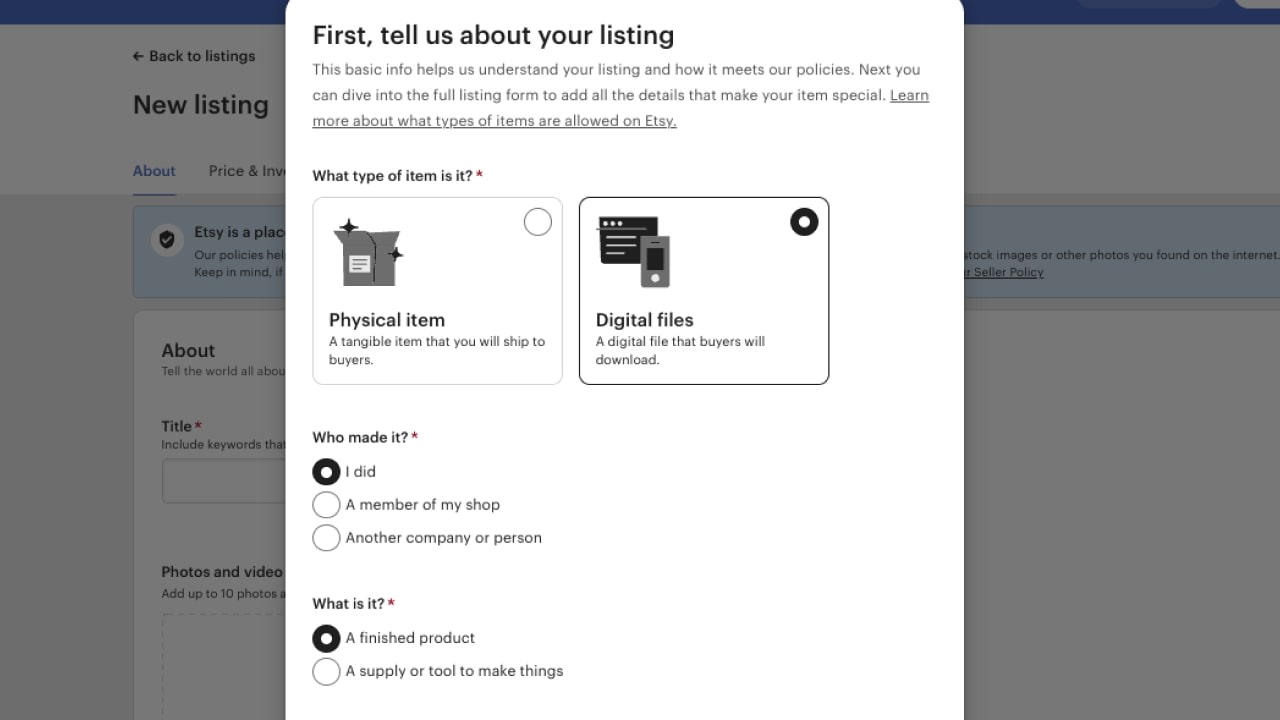The image depicts a webpage interface with various sections and options. On the left, there is a grayed-out area with black text that reads "New Listings." Below, green text accompanied by an arrow pointing left says "Back to Settings." On the right side at the top, there is a blue bar.

Partially obstructing the page is a white pop-up with black text, explaining the initial steps in the listing process on Etsy. The text reads, "First, tell us about your listing. This basic info helps us understand your listing and how it meets our policies. Next, you can dive into the full listing form to add all the details that make your item special." Below this, an underlined prompt states, "Learn more about what types of items are allowed on Etsy."

The form within the pop-up prompts the user to specify the type of item. Options include "Physical Item" and "Digital Files," with the latter selected. It then asks, "Who made it?" with selectable options being "I did" (selected), "A member of my shop," and "Another company or person." It further inquires, "What is it?" with options like "A finished product" (selected) or "A supply or tool to make things."

Scattered across the interface are titles and headings such as "Title," "Photo and Video," "Price" (which might be a placeholder given the apparent typo "V," likely meant to be "Invoice"), "Etsy," and "About." The user seems to be in the early stages of filling out this form.

The message ends with a note of gratitude, saying, "Once again, thank you. Back to you and your team for all these. It's been fantastic. Thank you very much to you and your team. Hopefully, do this again soon."